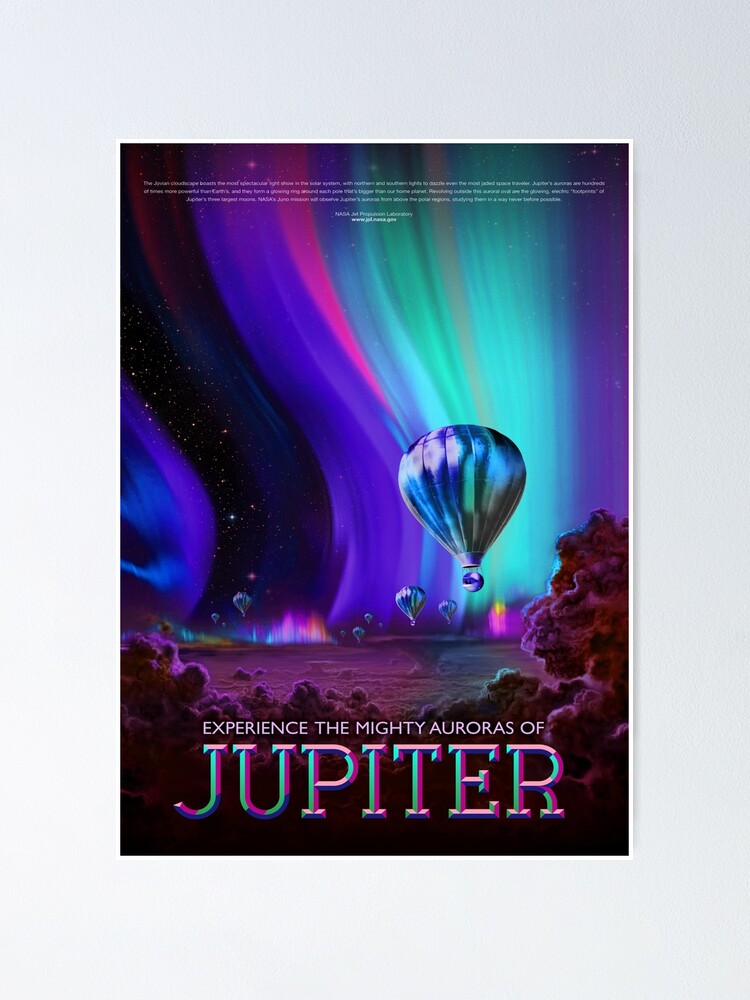The poster from NASA's Jet Propulsion Laboratory vividly captures the majestic spectacle, urging viewers to "Experience the Mighty Auroras of Jupiter" in bold, colorful letters at the bottom. The captivating sky, reminiscent of Earth's northern lights, is awash with brilliant hues of blue, purple, pink, green, and turquoise. Twinkling stars and puffs of blue smoke add depth to the celestial panorama. Hot air balloons in various shiny colors float through this luminous scene, with a prominent blue and green balloon in the foreground reflecting the auroras' mesmerizing glow. Smaller balloons dot the distant sky, appearing tiny against the vastness. Beneath this vibrant display, the landscape features clusters of crater-like purple rocks, adding a surreal touch to the picture. At the top, additional text appears in tiny white font, blending into the enchanting atmosphere. This breathtaking portrayal masterfully combines elements of science and art, showcasing the awe-inspiring beauty of Jupiter's auroras.